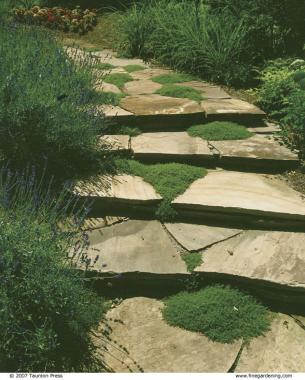The photograph depicts a weathered stone stairway located outdoors, bordered by abundant vegetation. The stairway consists of five shallow steps, each formed by several slate pieces, which have become worn and flattened over time from frequent use. Moss and various plants, including lavender on the left and unidentified ferns on the right, have found their way into the crevices and cracks of these steps, accentuating the natural decay and long-standing presence of the stairway. The steps lead to a meandering stone pathway that vanishes into the distance, surrounded by greenery and hints of flowers, particularly on the upper left side. The overall ambiance created by the slate gray of the stones contrasted with the vivid greens of the surrounding plants and moss suggests an area that has gracefully aged within its natural setting.